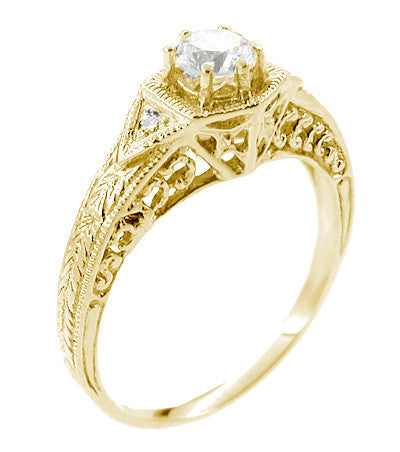This detailed product image showcases an ornate gold engagement ring set against a stark white background. The ring, floating and slightly angled, reveals a large central diamond secured by six prongs. The band is meticulously crafted with intricate sculpting that features swirling floral and leaf-like patterns, complemented by feather-like designs extending down the sides. The lattice-like etchings, adorned with semicircles and S-shaped curves, enhance the ring's intricate aesthetic. Flanking the central diamond, smaller diamonds are nestled within triangular gold settings, adding to the ring's opulence. The bright yellow gold and clear, sparkling diamonds highlight the ring's luxurious and elegant design.